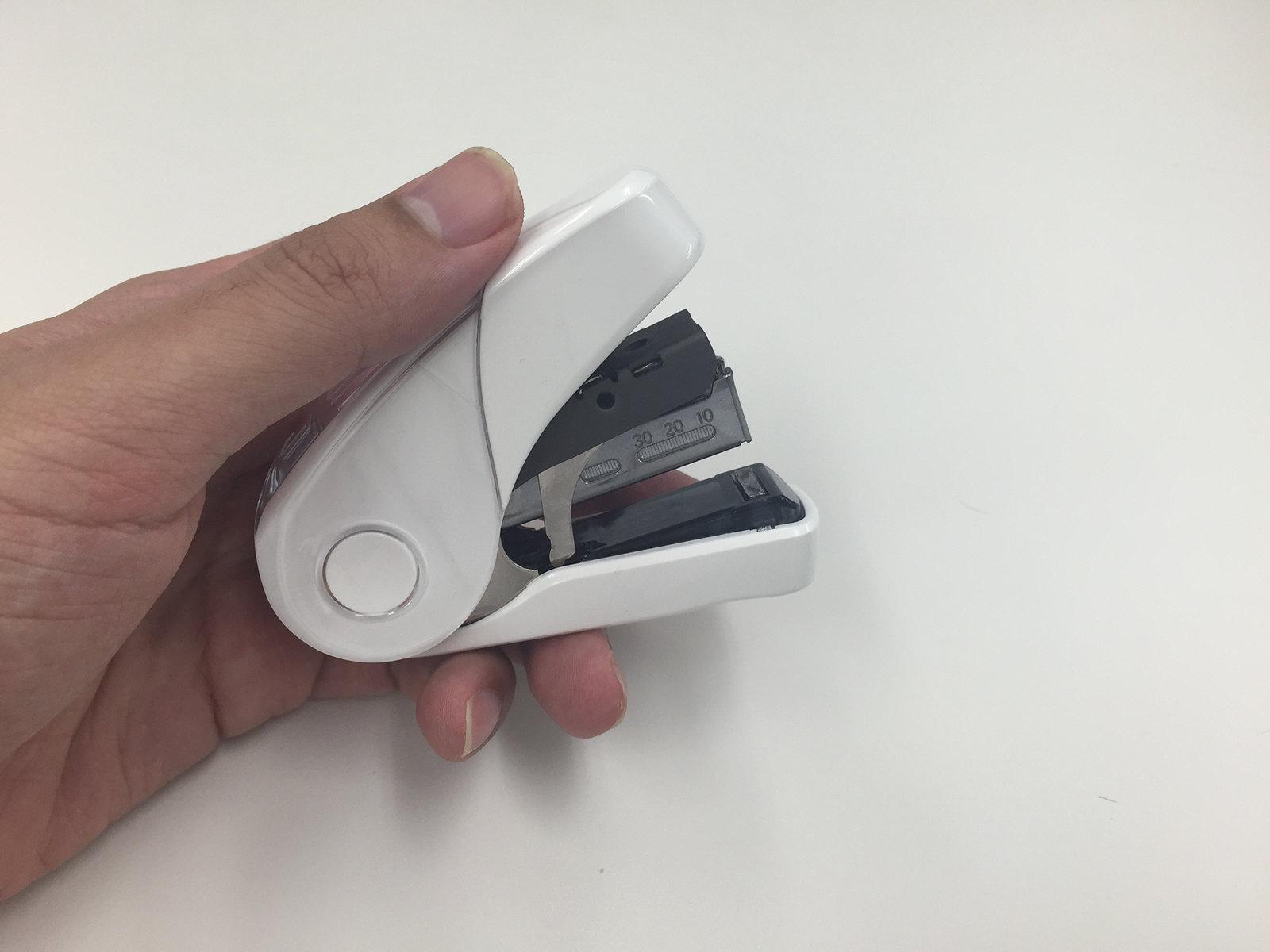In this close-up image, we see a person's left hand holding a very small, white mini stapler. The hand, with detailed fingernails and visible cuticles, extends from the left side of the frame against a pristine white background. The stapler is distinguished by a white plastic exterior, alongside a silver metal mechanism in the center that bears the numbers 10, 20, and 30. The stapling mechanism, ready for action under the person's thumb, includes a visible gray rectangle and a designated slot for staples which appears to be filled. The structure of the stapler features a black plastic component and a circular white joint at the back, ensuring its compact and functional design. A subtle shadow from the hand and stapler is cast below, enhancing the depth of the image.